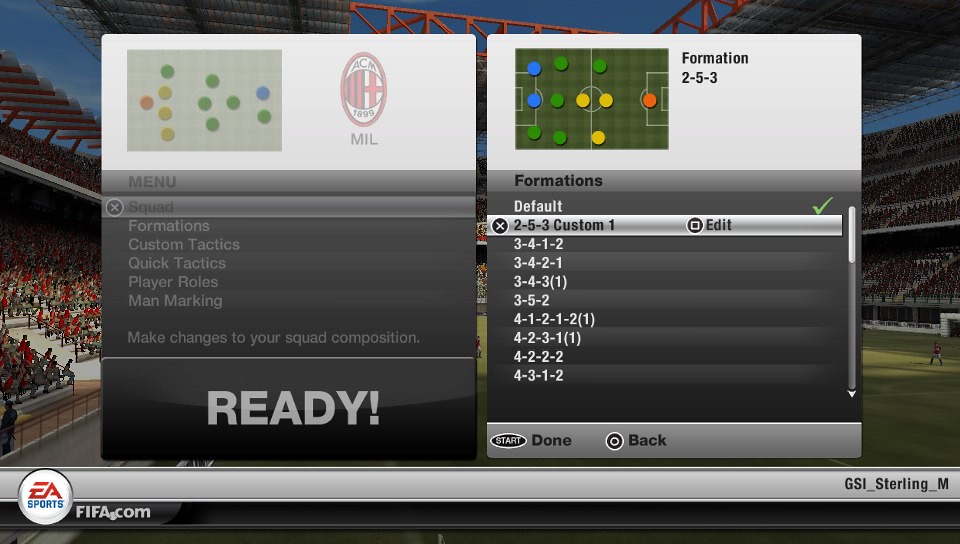The image is a detailed screenshot from the FIFA EA Sports video game on a computer screen. The background showcases a 3D-rendered soccer stadium filled with fans, predominantly dressed in red, cheering from the stands. The soccer field, lush and green, serves as the setting for the scene. In the foreground, two main interactive menu boxes dominate the screen.

The box on the left contains sections labeled "Squad," "Formations," "Custom Tactics," "Quick Tactics," "Player Roles," "Man Marking," and an option to make changes to squad composition. This menu also features a pixelated football field with multi-colored dots indicating player positions in various formations. Text such as the team insignia "ACM 1899," and "MIL" are prominently displayed. The section underscores player positioning, emphasizing formations such as 2-5-3.

To the right, another menu box shows specific formations and default settings for team layout, with options listed as "2-5-3," "3-4-1-2," "3-4-2-1," "3-4-3 (1)," "3-5-2," "4-1-2-1-2 (1)," "4-2-3-1 (1)," "4-2-2-2," and "4-3-1-2." At the bottom of this box, there are control options labeled "Start," "Done," and "Back," facilitating game setup.

A light gray horizontal banner at the bottom of the screen contains the EA Sports logo, "FIFA.com," and additional text elements. The words "Ready!" in bold font draw attention to the preparedness of the game setup. The meticulous detail in the menus, including numerical formation codes and player management options, highlights the sophistication and depth of the FIFA EA Sports gaming experience.